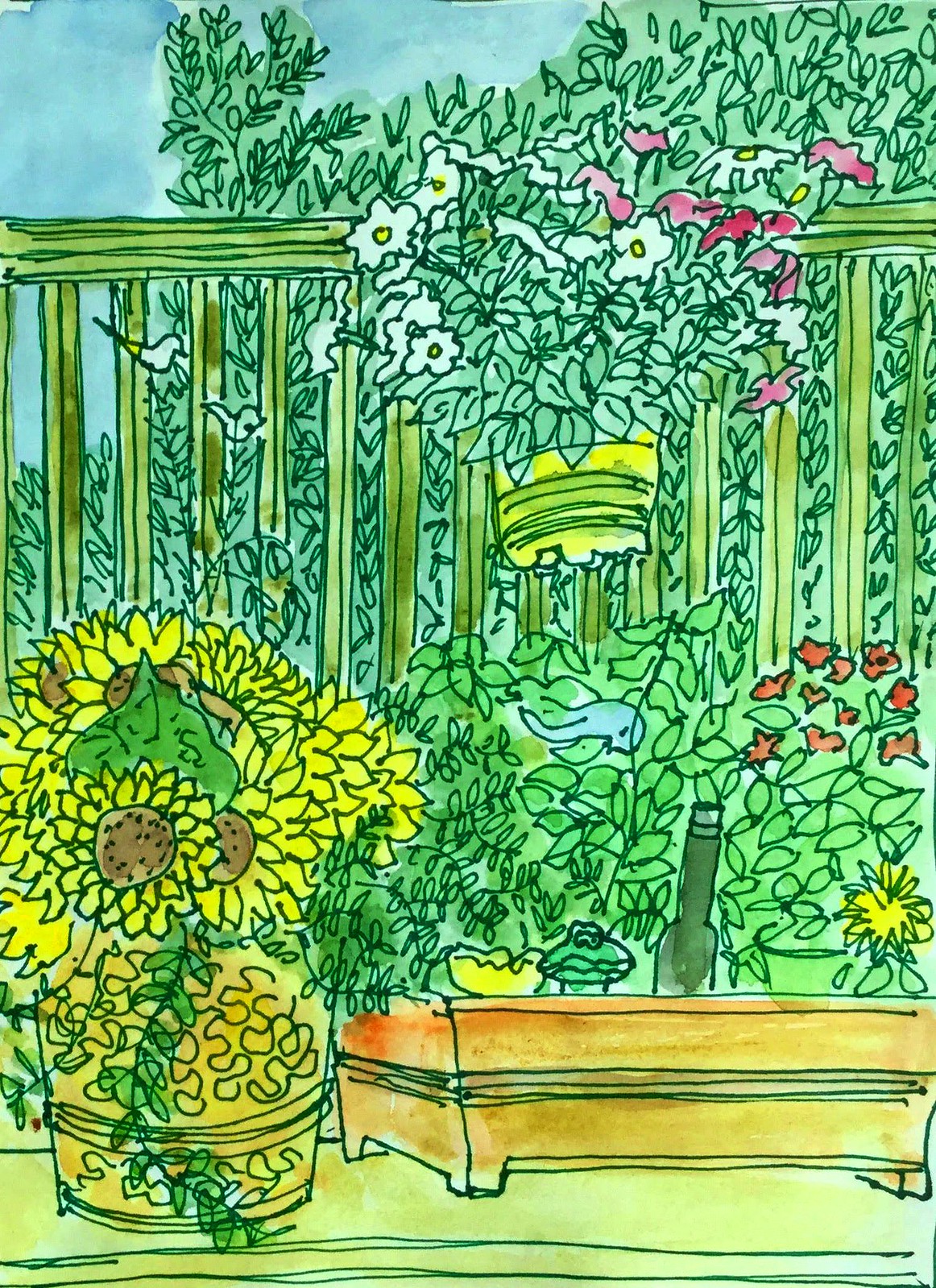This detailed caption describes a richly colored illustration, possibly sourced from a coloring book, rendered with precise lines in dark pen or pencil. The image depicts a serene garden scene featuring several distinct elements:

In the top left corner, a clear blue sky peeks through, accentuating the lush greenery of shrubs and trees that frame the garden. A verdant green fence runs horizontally, with a hanging pot plant secured to it. The pot, a yellowish-green hue, holds a cascade of vibrant white and pink flowers, interspersed with abundant green leaves.

In the lower left-hand section, a cluster of sunflowers, showcasing their bright yellow petals and rich brown centers, is arranged in a vibrant, darker yellow vase. The vase is round with an intricate, squiggly design, complementing the flowers within.

Towards the middle-right, a wooden bench stands as a central feature. Atop the bench are several objects: a bottle, some fruits, and perhaps a smaller pot plant, adding to the garden's charm. Flanking the bench, more pot plants add splashes of color with their red and blue containers.

Completing the scene, the garden floor is a natural green, tying together the various elements in a harmonious and tranquil composition.